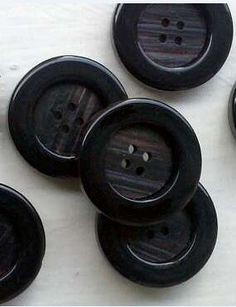The photograph displays a collection of black buttons arranged on a white, wood-like surface. There are five fully visible buttons in the foreground, with a hint of a sixth button peeking in from the right side of the image. The buttons are all identical, likely from the same garment, featuring a smooth black design. Each button has four holes in the middle for sewing, and a raised circular edge surrounding an indented center. The center of the buttons is banded with a multicolored pattern that includes shades of black, dark blue, light blue, and gray. On the left side, one button is partially visible, while three buttons in the center of the image overlap slightly. The outer edges of the buttons have a glossy, chrome-like finish that contrasts with the more matte and patterned inner section.